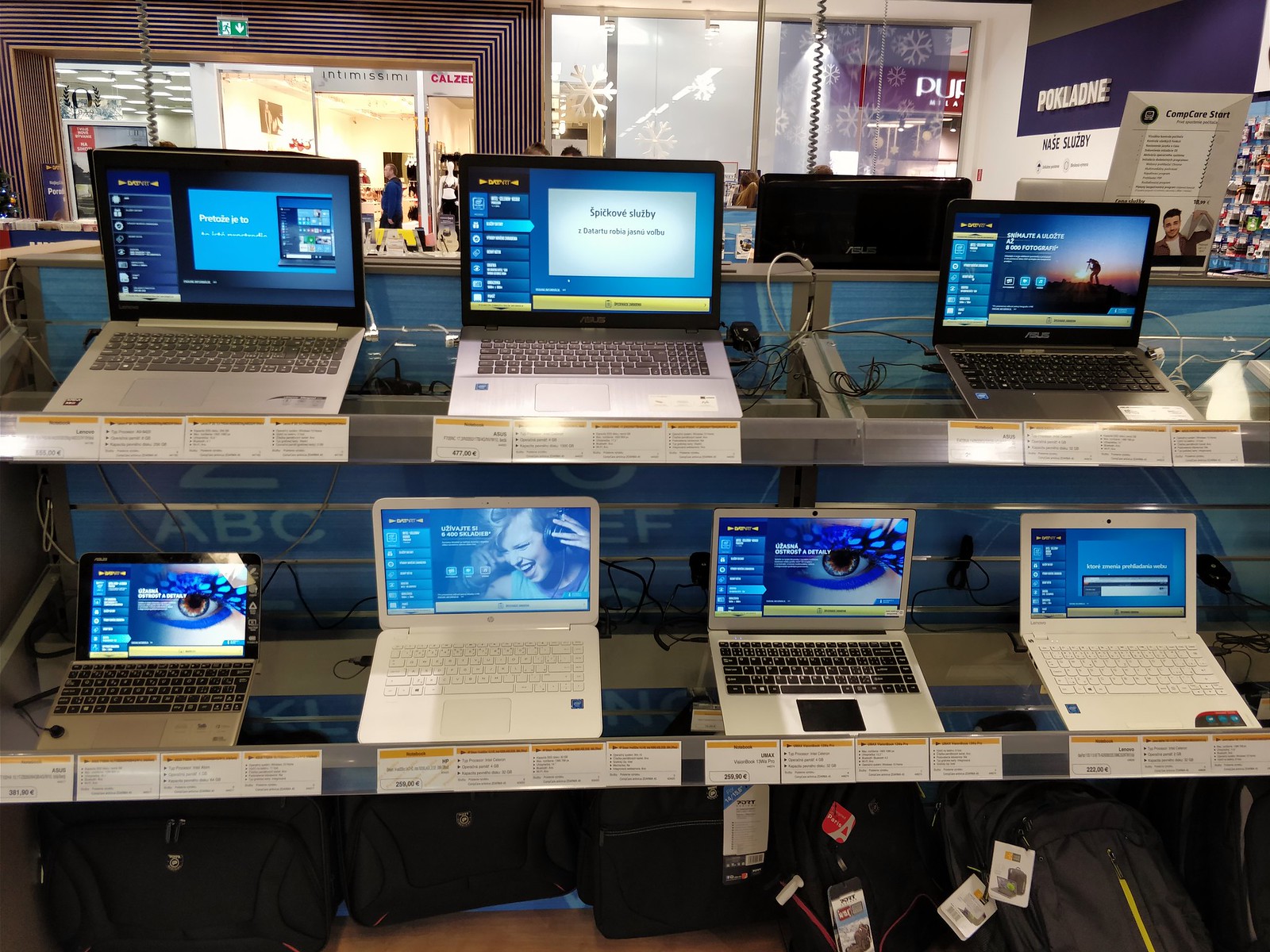The photograph captures a display of seven laptops on two shelves inside an electronics store, possibly a Best Buy. The top shelf features three laptops, while the bottom shelf holds four. All laptops are powered on, with their screens illuminated, and small white tags with yellow bands, likely indicating price and specifications, positioned in front of each. The laptops vary slightly in size and color, including white, black, and silver models. The scene extends beyond the immediate display, revealing a view through a plate glass window into the corridor of a mall. Opposite the store, you can see two storefronts, and to the right, part of another hallway and courtyard area. Below the bottom shelf, the image shows a dark brown floor cluttered with tags and debris, alongside black boxes—potentially laptop cases—stacked in a somewhat disorderly manner. The right side also features a partial view of a sign that reads "Pokladene."